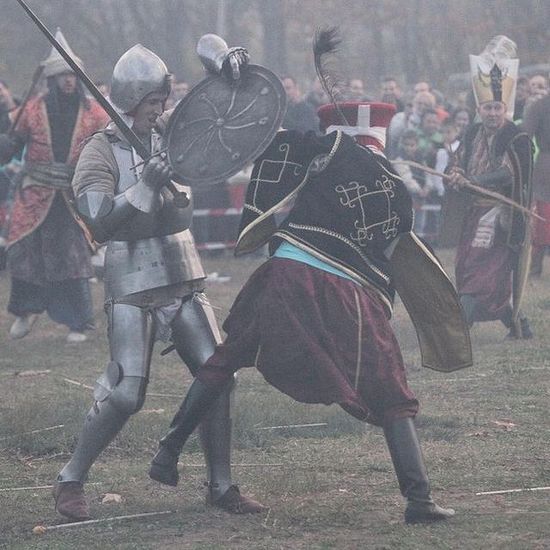In this image capturing a medieval battle reenactment, two men are engaged in a dramatic clash on a grassy field scattered with tan arrows. The man on the left is clad in a full suit of authentic-looking metal armor, wielding a sword and a metal shield, attempting to block a strike. His opponent on the right is flamboyantly dressed in a black velvet jacket with gold accents, a velvet skirt, black riding boots, and a red hat that resembles a crown. The red hat also features a feather and white accents. The background is bustling with figures dressed in a variety of medieval costumes, including one who looks like a samurai on the top left and another who resembles a bishop in a tall hat and robe on the top right, carrying a stick. Despite a gray, overcast sky lending a dull tint to the scene, the field is lively. A line of spectators can be seen behind a black, white, and red fence, watching the action unfold with keen interest. The foggy atmosphere and the detailed costumes contribute to the authentic and immersive experience of the reenactment.